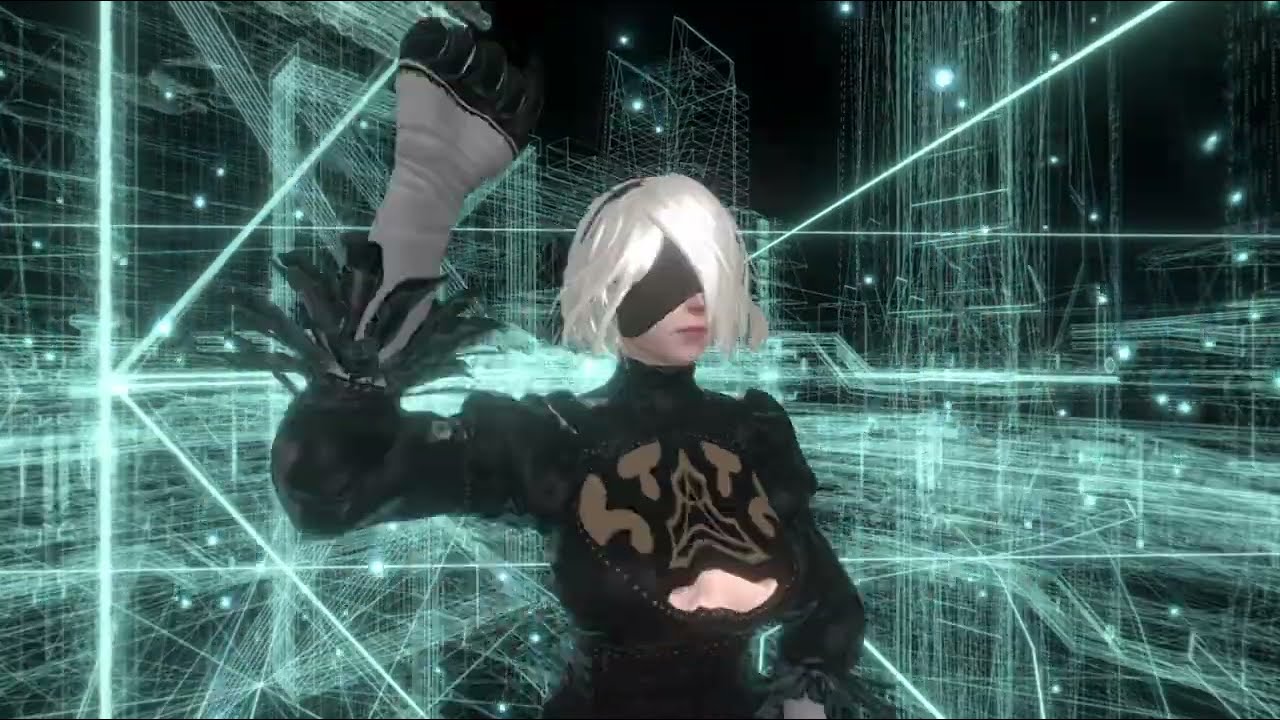The image is a highly detailed 3D rendering of 2B, a character from the popular video game Nier Automata. The character is depicted from the waist upwards. 2B has short, white, almost glowing hair, with a black headband, and her eyes are covered by a black cloth blindfold. She is wearing a distinctive black blouse that features a window displaying her cleavage, and her sleeves end in black feathers. Her left hand rests at her waist, while her right hand is raised in a fist above her head, adorned in a white glove with black fingers. The background is a complex array of green lines forming square and rectangular structures, giving a futuristic, cyberspace-like ambiance akin to something from the Tron universe.